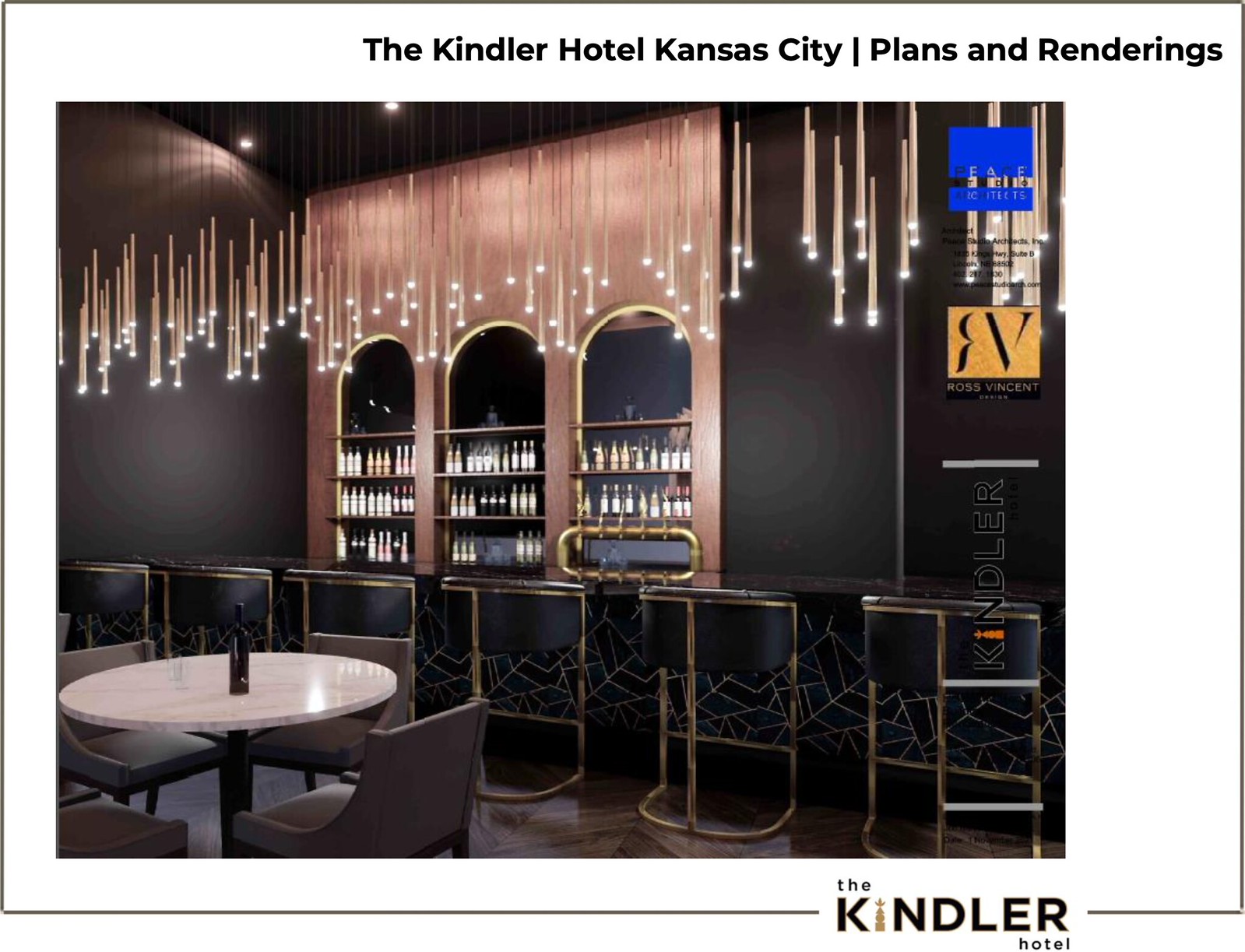This advertisement showcases the interior of the Kindler Hotel in Kansas City. The image is framed by a thin black border within a white rectangle, and at the top in black lettering, it reads "The Kindler Hotel, Kansas City, Plans and Renderings." Beneath this header lies an intricate depiction of the hotel's modern Regency-style bar. The bar features a sleek, dark counter adorned with round, gold-trimmed black bar stools. Above the bar, hundreds of lights hang from the ceiling on thin cables, resembling floating candlesticks that create a stunning luminescent effect. The backlit bar itself is a triple archway design, presenting neatly organized rows of liqueurs and alcohols against a soft rose-gold shelving and dark brown wood. In the background, there are smaller white circular tables surrounded by chairs, with a bottle of alcohol placed on one of them. An overlay panel on the right side of the image contains information about the hotel, mentioning names like Kindler, Ross Vincent, and Peace Studio Architects. The overall setting is meticulously clean and exudes a classy and sophisticated ambiance. At the bottom of the image, the Kindler Hotel name appears once more.